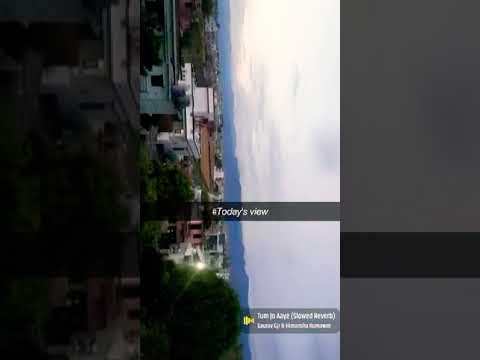The image appears to be a TikTok video, taken vertically but displayed sideways, showing a cityscape likely viewed from the balcony of a hotel or similar high vantage point. The scene captures an older city or small village with buildings that appear to date back to the 1930s or 1940s. The architecture includes white houses with dark gray rooftops, complemented by green trees. Apartment buildings and possibly other hotels can be observed, with the ocean visible beyond the cityscape. The sky above is cloudy, contributing to a washed-out appearance in the photograph. There's a caption in white letters that reads "Today's View," positioned against a gray background. The lower part of the image includes another blurry text caption with a yellow icon next to it, though the exact wording isn't legible. The overall aesthetic features a mix of browns, whites, and blues, imbuing the scene with a blend of residential and architectural elements.